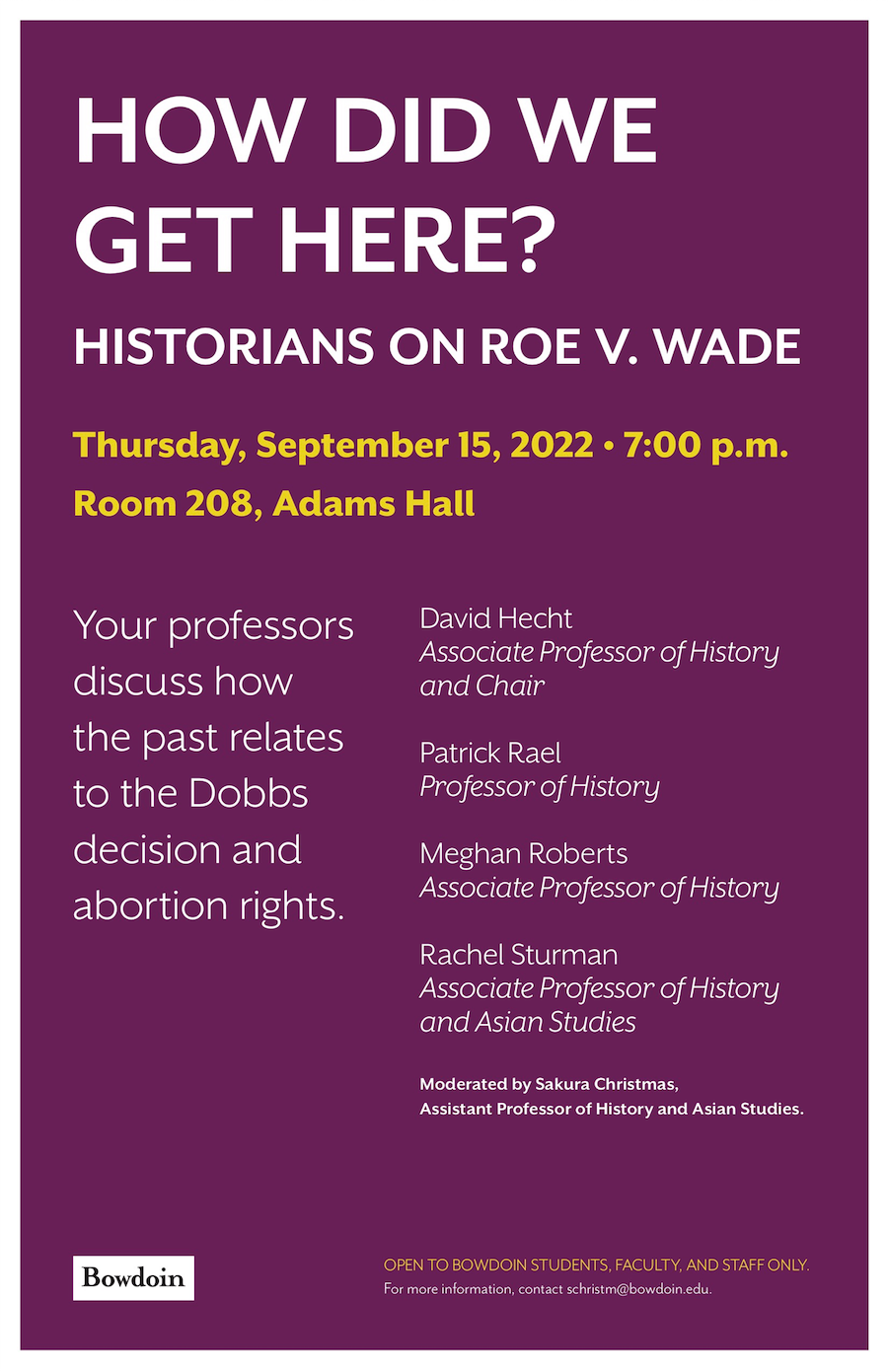This vertical, rectangular flyer features a purple background and is dedicated to the lecture titled "How Did We Get Here? Historians on Roe v. Wade." The title is prominently displayed at the top in white, all capital letters. Below the title, the event details are in yellow: "Thursday, September 15, 2022, 7 p.m., Room 208, Adams Hall." On the left-hand side, the flyer includes a paragraph in white text explaining, "Your professors discuss how the past relates to the Dobbs decision and abortion rights."

On the right-hand side, four professors are listed: David Hecht, Associate Professor of History and Chair; Patrick Ryll, Professor of History; Meghann Roberts, Associate Professor of History; and Rachel Sturman, Associate Professor of History and Asian Studies. The event is moderated by Sakura Christmas, Assistant Professor of History and Asian Studies. The flyer also notes that the event is "open to Bowdoin students, faculty, and staff only" in very small script below the moderator's information. Additionally, a small white rectangle at the bottom left corner contains the word "Bowdoin."